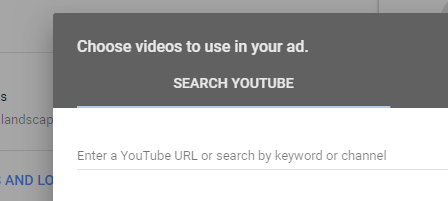This image is a screenshot featuring a partially visible background with a grayed-out area. The background text appears slightly pixelated and contains fragments of the word "landscaping" and a partial blue text saying "LO." Overlaying the background is a prominent dark gray and white box. At the top of this box is a dark gray bar with light gray text that reads, "Choose videos to use in your ad." Following this, in all caps, it says "SEARCH YOUTUBE." Beneath this is an ultra-thin white pull bar.

The main section of the overlay has a white background with gray text instructing users to "Enter a YouTube URL or search by keyword or channel." Underneath this instruction, there is a thin gray line. The overlay is presented in high quality with large, easy-to-read text, containing no color bleeding or extra images. The overall design is straightforward, ensuring clarity and ease of understanding.